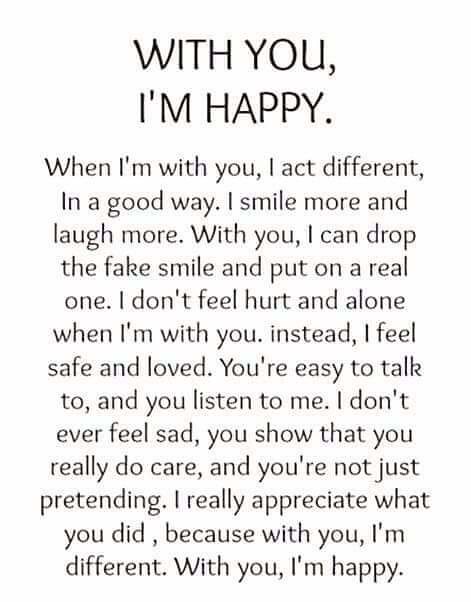The image features a black sans-serif text on a white background, presented in portrait orientation. The heading, in all caps, reads "WITH YOU, I'M HAPPY." Underneath this title, a centered and stylistically modern paragraph unfolds, expressing heartfelt sentiments. It starts with, "When I'm with you, I act different in a good way. I smile more and laugh more. With you, I can drop the fake smile and put on a real one. I don't feel hurt and alone when I'm with you. Instead, I feel safe and loved. You're easy to talk to and you listen to me. I don't ever feel sad. You show that you really do care and you're not just pretending. I really appreciate what you did because with you, I'm different. With you, I'm happy." This touching, romantic statement reflects genuine affection and appreciation.